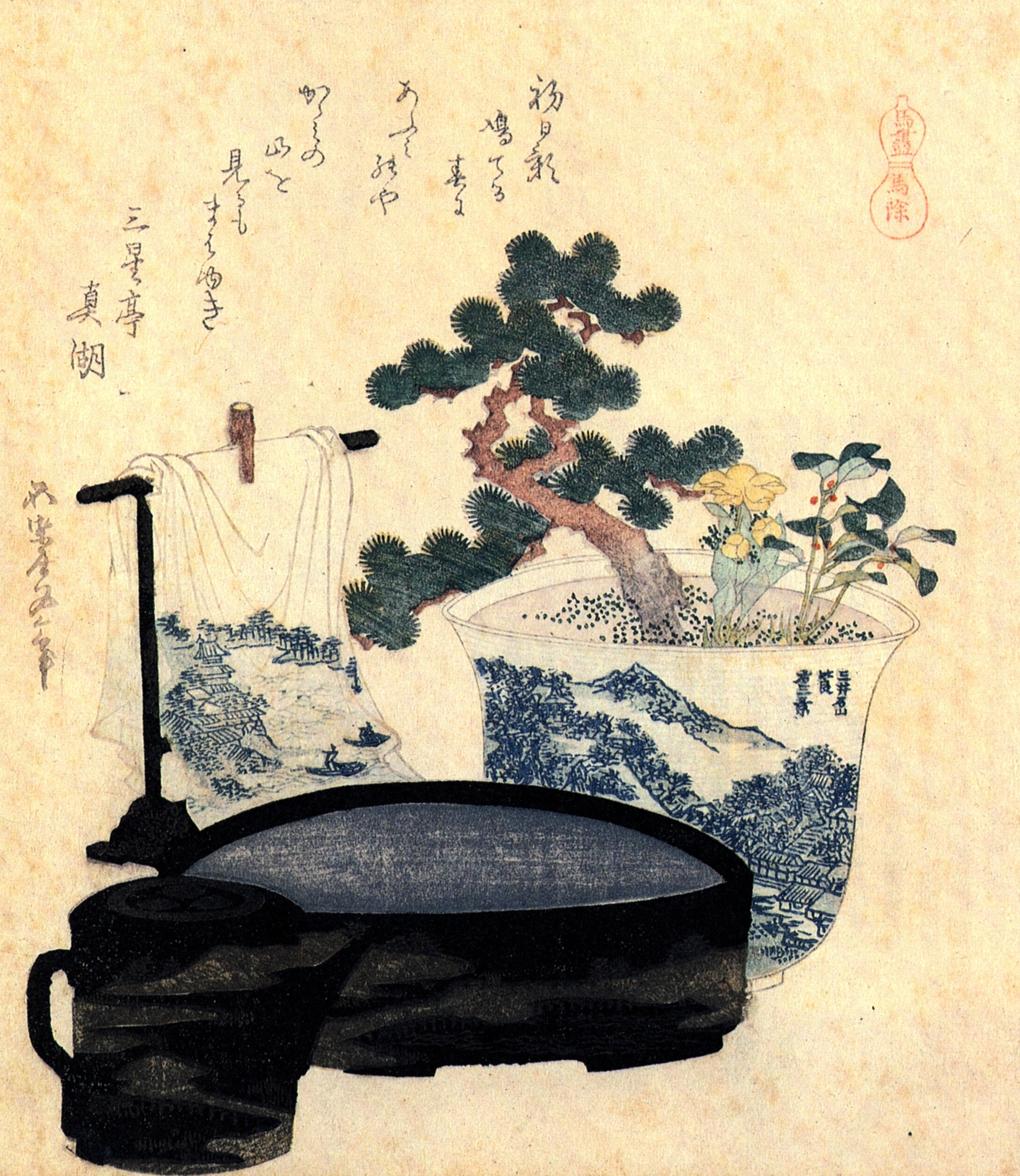This is a vertically aligned rectangular drawing set against a pinkish-brown background, with a texture resembling parchment or linen. Brown spots mark the top, but the overall hue is predominantly pink. Vertical black Asian script adorns the upper left, and the upper right features additional writing in red, reminiscent of a watermark.

In the foreground, there is a circular water basin, predominantly black and gray on its outer side and dark blue and white within. To its left, a simple black mug with a handle is positioned, and nearby, a teapot with a black handle and shading in black and gray is vaguely noticeable.

Dominating the center of the drawing is a large, ornately detailed white pot. This pot displays blue vertical symbols and intricate illustrations of mountains, a hillside, and a village. Within the pot, black dots signify soil. From the soil springs a diverse array of plants: on the right, thin stems with dark green leaves and red berries; in the middle, light green leaves with yellow flowers; and on the left, a thicker brown branch bearing spiky, round black shrubs, suggestive of a juniper plant. Together, these elements create a harmonious and detailed Japanese-style painting.